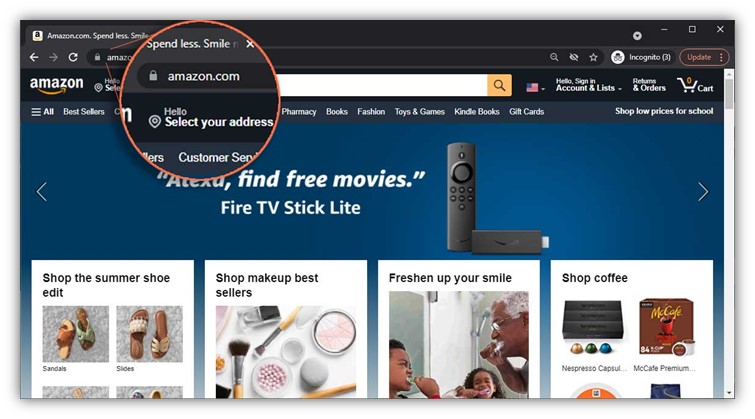The image features a dark blue background with a prominent black box at the top displaying the text "Amazon.com" accompanied by the signature Amazon smile logo. Adjacent to this is a left arrow with the text "Spend less, smile more". The "Amazon.com" text and "Hello, select your address" are circled in red for emphasis. 

To the right, there is a series of navigation options including "Customer Service," a large search box, an American flag for international settings, "Account & Lists," "Returns & Orders," and a shopping cart icon. Below these, there are three horizontal lines indicating a menu with categories like "All," "Best Sellers," "Books," "Fashion," "Toys & Games," "Gift Cards," and "Low Prices for School."

Further down, another section with a blue background features a left arrow with the text "Alexa, find free movies," followed by icons for the Fire TV Stick Lite and its remote control, and a right arrow. 

At the bottom of the image, there are four pictures against a white background, each with its own shopping category: “Shop Summer Shoe Edit,” “Shop Makeup Bestsellers,” “Freshen Your Smile,” and “Shop Coffee.”